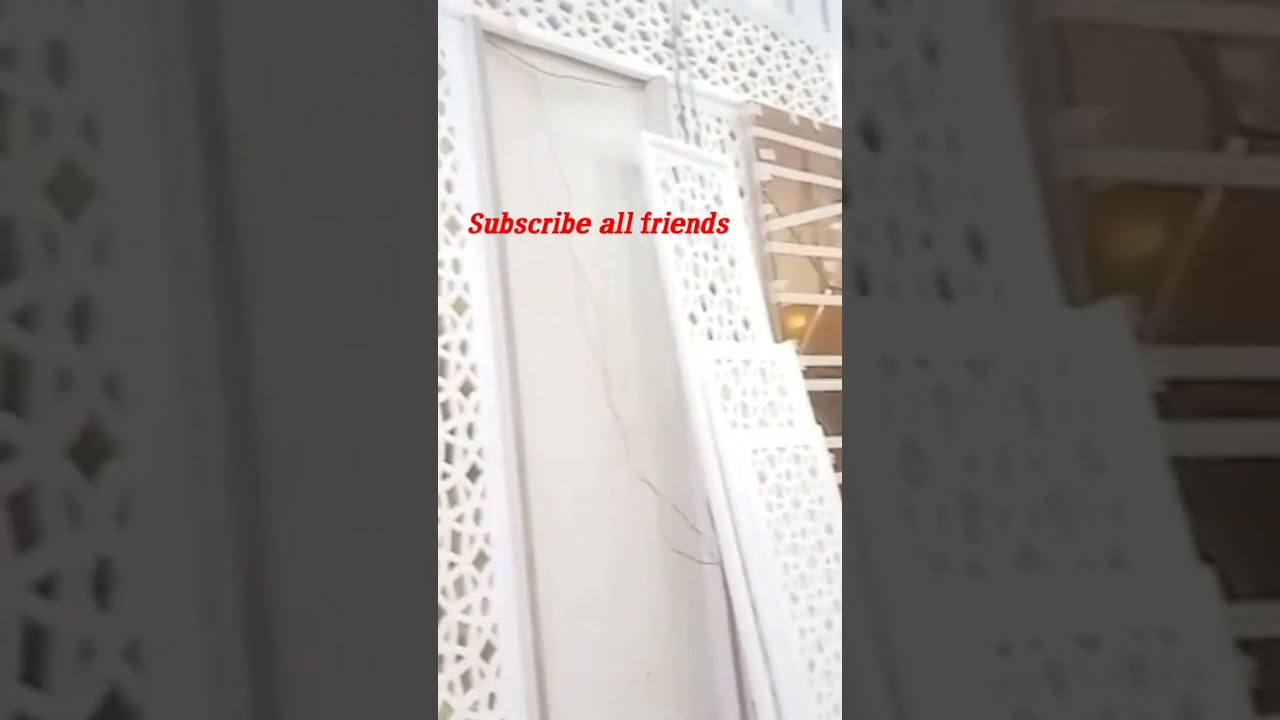The image is divided into three sections. The central section, which is brightly lit, features a white lattice pattern on a wall with a large doorway cut out. Some areas lack the lattice, showing only horizontal boards, seemingly unfinished. Overlaid in bold dark red font, the text "subscribe all friends" is prominently displayed. On the left and right sides are zoomed-in fragments of the central section under darker lighting. The left side closely examines the lattice work and the boards, while the right side offers a closer look at the unfinished spaces near the doorway. The overall impression is of an in-progress construction, possibly a partition with a laser-printed pattern between rooms. The repeating text underscores a likely call to action related to a video tutorial or DIY project involving tools and materials.